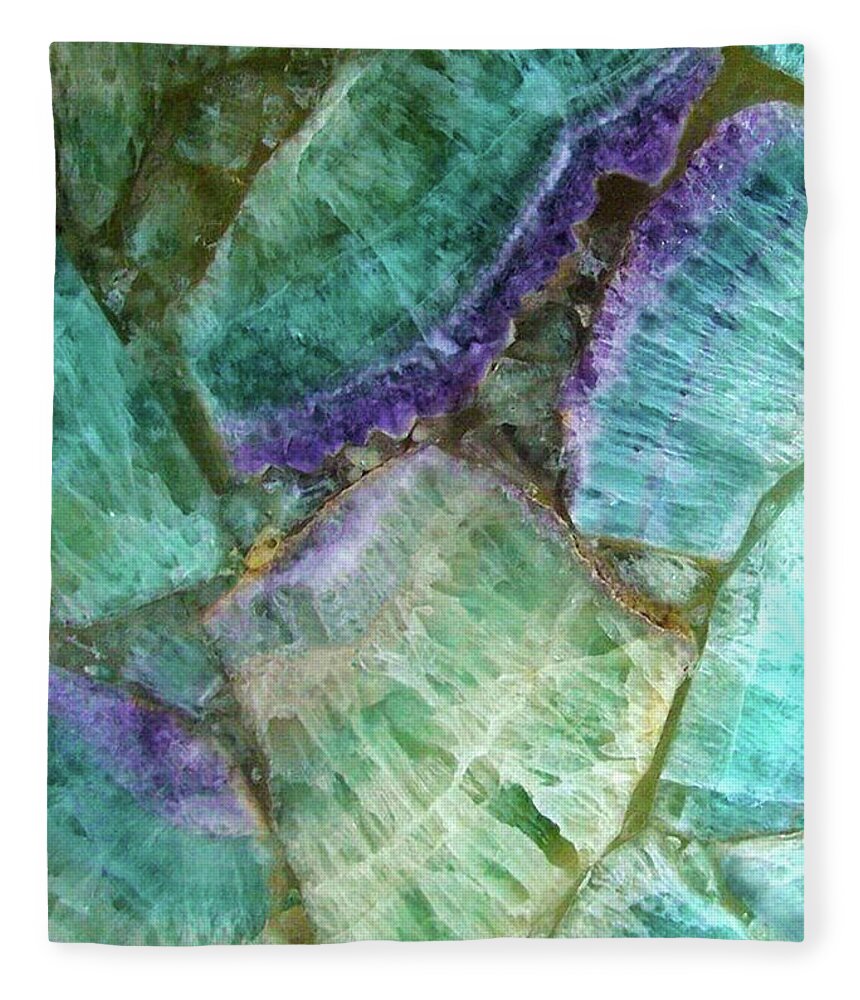This color photograph is a detailed close-up of a segmented piece of fluorite mineral. The image showcases numerous pieces, approximately half a dozen, exhibiting a stunning array of colors including hues of turquoise, green, blue, and purple. The sections are visually separated by brown-green seams, with some segments displaying intricate white veins that run vertically through them. The largest central piece is green with white stripes, surrounded by segments ranging from bright purple to a purple similar to amethyst, and areas with beige or brown tinges. The mineral appears polished or in the process of being polished, highlighting the beautiful, varied patterns and layers within the rock. The intricate lines and color variations in the fluorite evoke the appearance of pineapple slices, where the lines radiate through the colored segments.